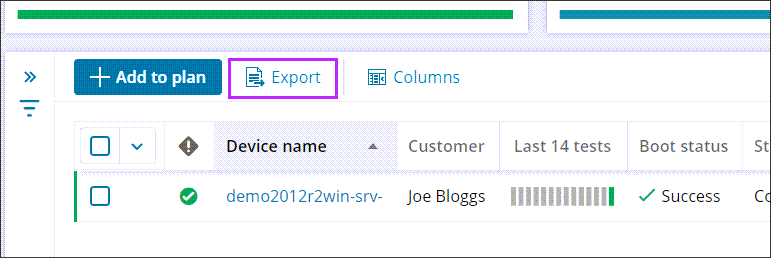This screenshot captures a detailed view of a window, featuring a UI layout for monitoring various device statuses and tests. At the very top, a green stripe is adjacent to a blue stripe, followed by a blue "Add to Plan" button and an "Export" button encased in a purple box. Next to these buttons is a Columns icon.

The main content area displays a chart with four columns labeled: Device Name, Customer, Last 14 Tests, and Boot Status. Below this, there is an entry where the Device Name is "DEMO-2012R2-WIN-SRV," Customer is "Jooblogs," Last 14 Tests visualizes a series of gray bars with the last bar colored green, indicating recent success. The Boot Status column shows a green checkmark labeled "Success."

To the far left of this entry, a checkbox remains unchecked. The page's background is predominantly white, with a disclaimer tag situated to the left of the Device Name column. The Device Name itself is highlighted in a lilac color, while the rest of the tabs and text are rendered in a standard white background with black text.